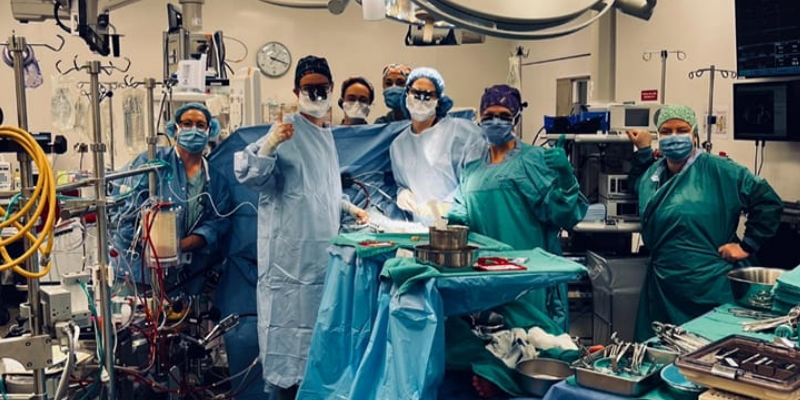In an operating room filled with medical equipment, a team of seven medical personnel, including doctors and nurses, all dressed in scrubs, hats, masks, glasses, and goggles, are gathered around a surgical table. The table, covered in a light blue cloth, seems to have a patient on it, although the focus is on the team rather than the procedure. Stainless steel tables bearing various surgical instruments and bowls are prominently displayed in the foreground. 

The room is well-lit with fluorescent lights overhead, and the background is cluttered with medical equipment such as IV poles and a yellow hose on the left edge of the image. A white clock is visible on the wall. The primary focus is the medical team, who have paused their work to face the camera, with the lead surgeon giving a thumbs-up. A hint of blood is visible on the surgeon's gloves. The scene is accentuated by the range of colors visible, including light blue, green, off-white, black, yellow, red, dark blue, and gray. This moment captures the intensity and camaraderie of a surgical team in action.